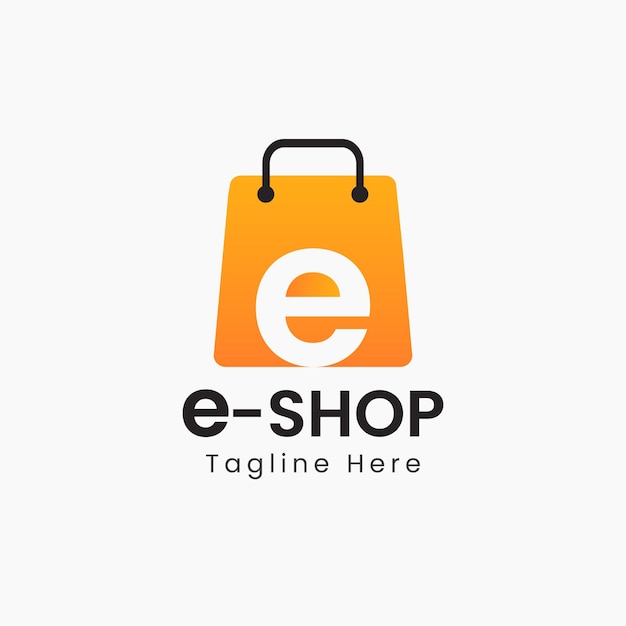The image showcases a logo on a square, light gray background. At the center is a minimalist depiction of an orange shopping bag that narrows slightly towards the top. The bag's color gradient shifts from a deep orange at the bottom to a lighter orange or yellow at the top. A curved black line with circles at both ends represents the handle, making it resemble a shopping bag. Inside the bag, centered at the bottom, there is a large, lowercase white letter "e". Beneath the logo, two lines of black text read as follows: the first line says "e-shop" with "e" in lowercase and "SHOP" in uppercase letters, while the second line, in smaller print, reads "tagline here".